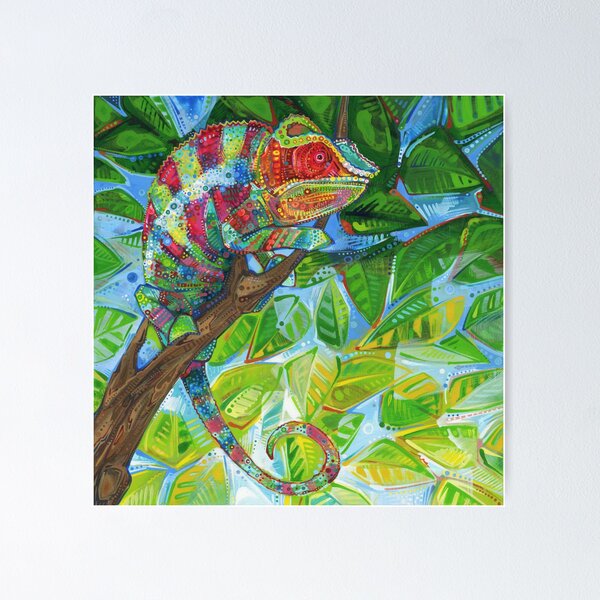This vibrant artwork depicts a multicolored chameleon on a textured brown tree branch that stretches diagonally from the left bottom corner to nearly the right bottom corner. The chameleon, with a tail wrapping in a circular shape beneath the branch, exhibits a mosaic of color blocks—its body adorned in vivid reds, greens, blues, and yellows. Its head stands out with a striking blue, while the sides of its face blend reds, oranges, and yellows, highlighted by an open mouth. The background features a sectioned color palette, transitioning from darker hues at the top to lighter shades towards the bottom. Surrounding the chameleon and filling the scene are intricately detailed leaves with visible veins, varying from darker tones above to lighter greens and pale yellows below. The pale blue sky provides a soft backdrop, enhancing the piece's vibrant and tropical aesthetic, bordered by a thin white frame that adds a subtle yet elegant touch.